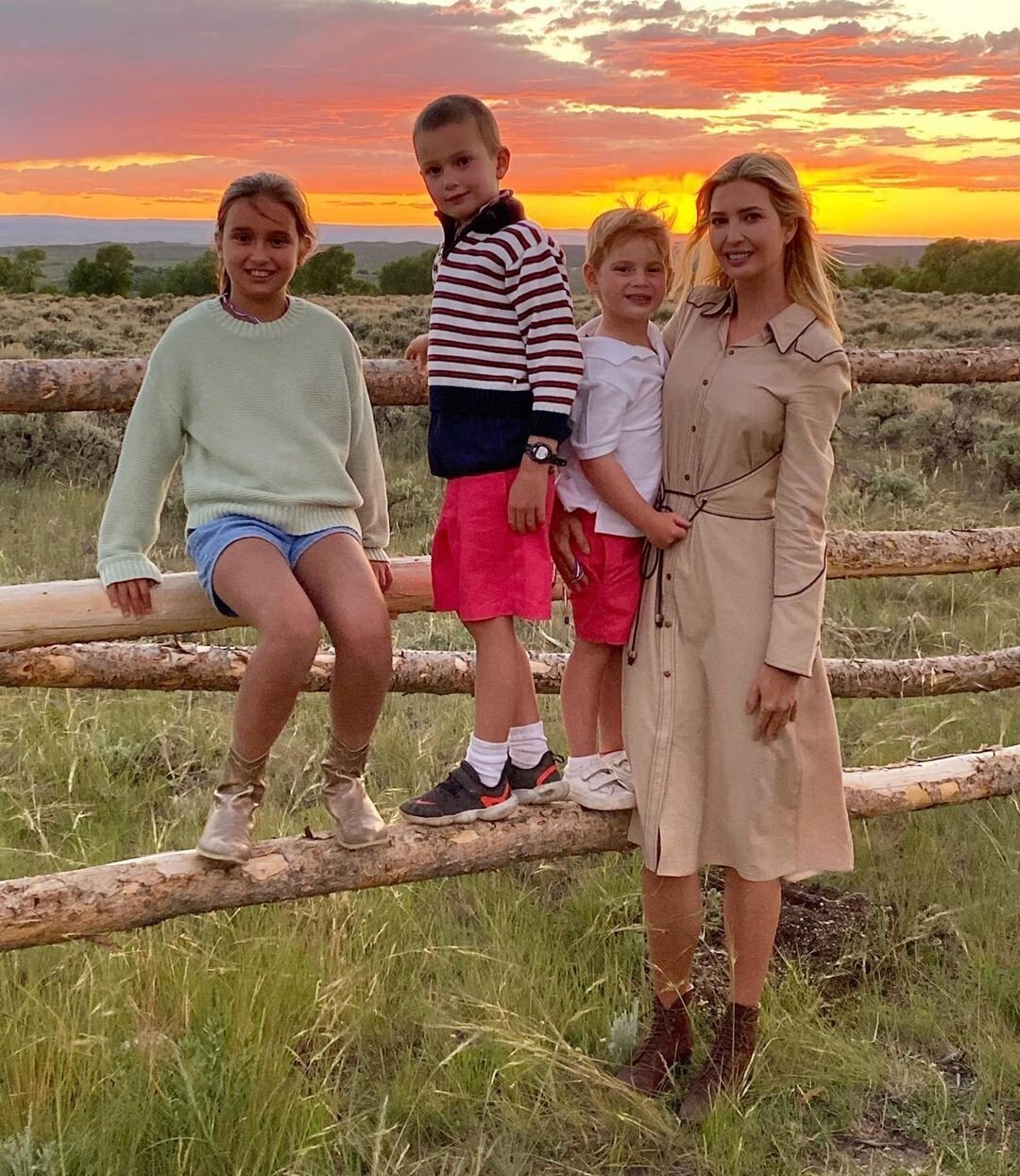This is a detailed image of a family of four – a mother and her three children – standing in front of a rustic log fence in a field. The adult woman on the far right is wearing a long-sleeved, knee-length beige dress with contrasting piping and brown boots. She has long, straight blonde hair parted down the middle and is smiling warmly with her arm around a small boy to her left. The small boy, who has blonde short hair, is standing on the bottom log of the fence. He is dressed in a white polo shirt, red shorts, and white shoes. 

To his left is an older boy with very short brown hair, wearing a black and white striped shirt, red shorts, and black shoes. He is also standing on the logs. Further left, the oldest child, a young girl with long brown hair pulled back, is sitting on one of the horizontal logs. She is wearing a light green sweatshirt and blue shorts. 

Behind them, the wooden fence is constructed from horizontal tree branches or logs, and the area is surrounded by tall grass. The picturesque background features a field transitioning into green trees and hills, capped by a stunning sunset with colors that shift from gray to coral and yellow as they reach the horizon. The entire family is smiling, encapsulating a cheerful and serene moment.